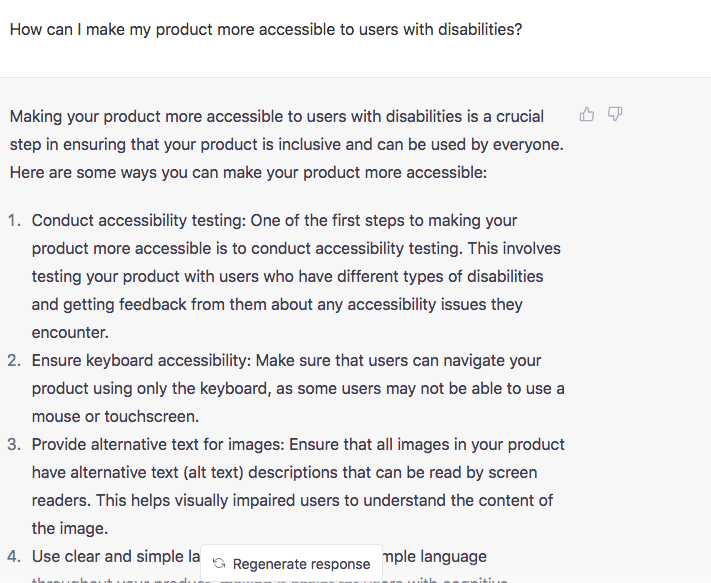**Detailed Caption:**

This screenshot, taken from a digital device (desktop, laptop, smartphone, or tablet), features a user interface aimed at aiding accessibility improvements for products. The background is a light gray, and prominently displayed in bold black text at the top is the question: "How can I make my product more accessible to users with disabilities?" 

Below this header, in mid-gray background, spans detailed information in black text. The section begins with an important introductory statement in bold black: "Making your product more accessible to users with disabilities is a crucial step in ensuring that your product is inclusive and can be used by everyone. Here are some ways you can make your product more accessible."

Alongside this text, the right-hand side displays thumbs-up and thumbs-down icons for user feedback. The content outlines accessibility tips, starting with:

1. **Conduct Accessibility Testing**: One of the initial steps to making your product more accessible is to conduct accessibility testing. This entails evaluating your product with users having different types of disabilities, and collecting feedback on any accessibility challenges they face.
  
2. **Ensure Keyboard Accessibility**: Guarantee that users can navigate your product solely using the keyboard, as certain users might not be able to use a mouse or touchscreen.
  
3. **Provide Alternative Text for Images**: Make sure all images in your product come with alternative text (alt text) descriptions that screen readers can interpret. This assists visually impaired users in understanding the image content.

The text continues with a partially visible fourth point: "Use clear and simple L-A...". Adjacent to this, a pop-up displays a light gray rectangle with a dark gray refresh symbol next to black text that reads "regenerate response." Outside the pop-up are the partially visible letters "N-P-L-E" in black text, indicating a continuation of the phrase "language" which is subsequently cut off.